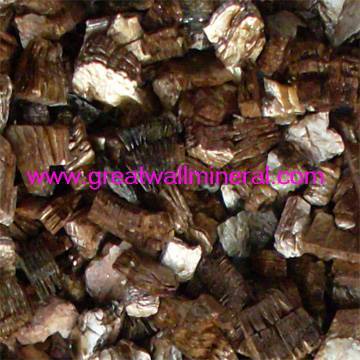The image showcases small, rectangular, square, and irregularly shaped rocks predominantly in shades of brown, with some appearing white and hints of brown, as well as a couple of pale pink ones on the bottom left corner. The rocks give a textured, uneven surface, filling the entire frame. On top of these rocks, somewhat centrally placed, is a website link – www.greatwallmineral.com – written in a pink or purplish hue. The image is notably zoomed in, resulting in a lack of crispness and visible digital artifacts. It's a close-up view that makes the stones, which resemble tiny candies or nuts in size, appear prominently detailed.